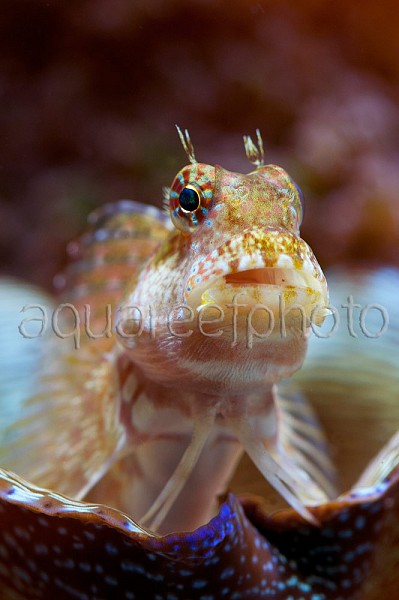This detailed close-up photo captures a distinctive marine creature, identified as an aqua fish or a sea amphibian, with unique and striking features. The creature is front-facing with large, black pupils encircled by intricate rings of alternating red and blue stripes. Adding to its vibrant appearance are the distinct, tan, pink, and dark yellow colors of its body, reminiscent of a glowing effect similar to LED lights. The fish sports a snail-like, gill-adorned body, while an elongated fin runs down its back and sides. Additionally, antenna-like fins are situated above both of its eyes, contributing to its exotic look. The open mouth of the creature, devoid of teeth, faces forward, lending it a curious expression. The backdrop features a striking red and white piece of coral. A watermark reading "AQUALEEF photo" spans across the middle of the image, indicating the title of this captivating marine life photograph.